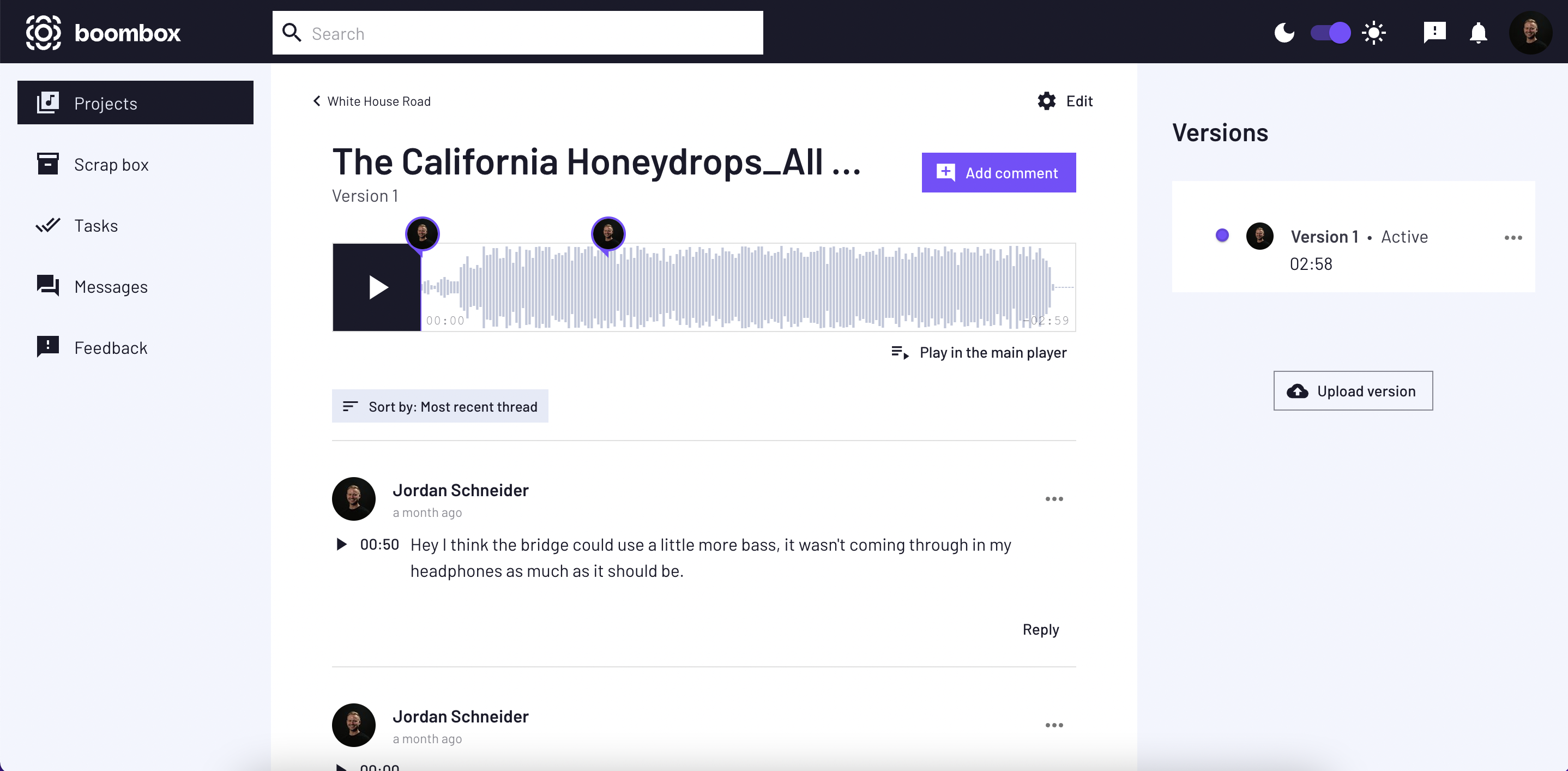This screenshot captures a detailed user interface of a music website named "Boombox." The top section features a black header with a white abstract flower icon on the top left, followed by the website's name "Boombox" in white text. Adjacent to the name is a white search bar with a gray magnifying glass icon on the left and placeholder text reading "Search" in light gray.

On the far right of the header are several icons: a white crescent moon icon, a purple toggle bar with a lighter purple circle on the right side (likely a theme switcher), a white sun icon, a white chat box icon housing a gray exclamation point, a white bell icon, and a user's profile picture.

The body of the website is structured with light gray sidebars on both the left and right, and a central section with a white background. In the top left of this central area, there is small gray text stating "White House Road" with a left-pointing arrow nearby. In the top right of the central section, a gray cog icon is labeled "Edit."

Below this section, large black text reads "the California honey drops underscore all..." To the right of this text, there is a purple button with white text saying "Add Comment," and to the left of this button, a white chat box icon with a purple plus sign inside. Beneath these elements, you'll find an audio waveform created with vertical gray lines. Adjacent to the waveform on the left side, there is a black square with a white right-pointing arrow, indicating a play button.